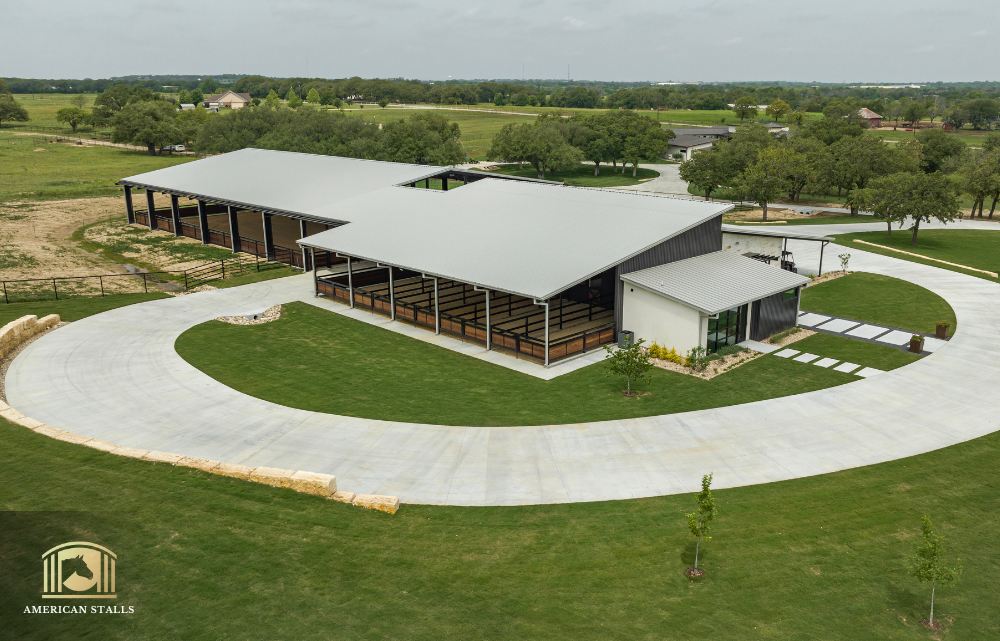This aerial image, likely taken from a helicopter or drone, offers a comprehensive view of a horse training facility named "American Stables." Situated in the bottom left corner is a notable arch adorned with alternating black and white bars. The arch frames a yellow background featuring a horse head outlined in black, looking right, with the text "American Stables" beneath it. Below the arch are two young trees exhibiting slender white trunks and sparse foliage, set against a vibrant green lawn. 

The focal point of the image is a large, covered structure identified as the main stables, characterized by multiple divisions designed to serve as enclosures for horses. These enclosures are open to the elements but feature bars that prevent animals from roaming freely. This stable region includes black fences encasing dirt paths and appears to have a functional design for horse training activities.

Encircling the stables is a broad, circular path composed of white rectangular stones leading to the building's entrance, which showcases a small, glass-windowed facade. On the left side of this circular area, portions of a yellow brick wall are visible. Extending from the circle's perimeter is an open, fenced-free area allowing additional space for horses to roam.

The property exhibits well-maintained grass in the foreground, while the background reveals patchier areas with visible dirt patches. Additionally, the scene includes several distant houses and is set against a grayish sky, completing the depiction of this equestrian training environment.